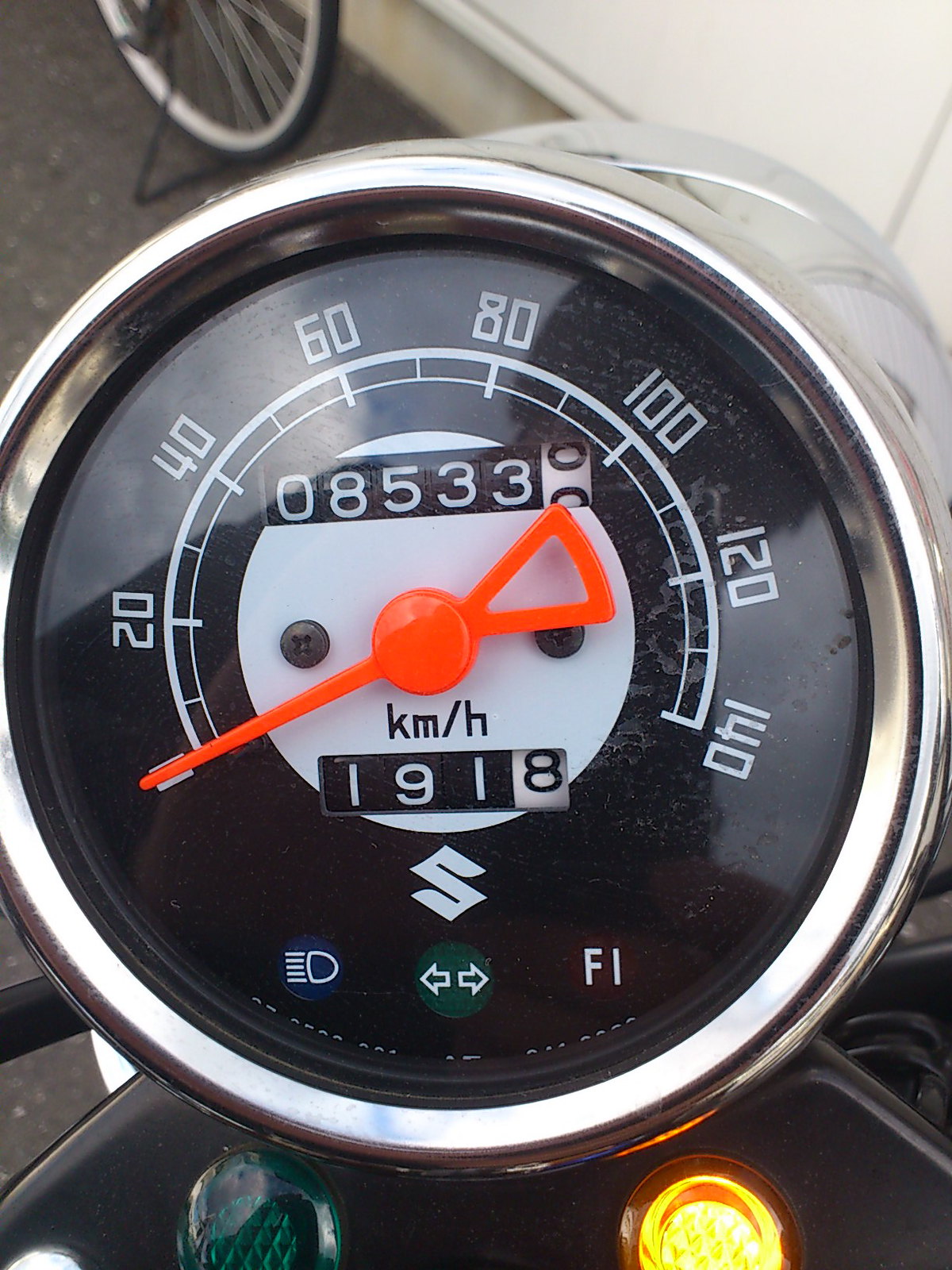In this detailed photo of a speedometer, the instrument is viewed from above, revealing its circular form. The outer rim of the speedometer is silver, encircling a black inner face. The entire device measures approximately seven inches in height and six inches in width.

At the center of the speedometer, there is a distinctive orange circle. From this circle, a short triangular pointer extends on one side, while a long orange needle stretches out to the opposite side, currently pointing all the way down to the left, indicating a speed of zero.

The speed readings are marked around the perimeter of the dial. Starting from the left and moving clockwise, the numbers read 20, 40, 60, 80, 100, 120, and finally 140 at the far right end.

In the middle of the speedometer, the numbers "08533" and "1918" are displayed, just above the text "KM/H" which denotes kilometers per hour. Beneath this section, there is a small green circle adorned with bi-directional arrows and the text "F1" adjacent to it. On the right side of this area, a bright yellow button is visible, while a darker green button can be seen on the left side.

This precise and complex arrangement of elements creates a clear, functional display for the vehicle's speed measurement and related information.